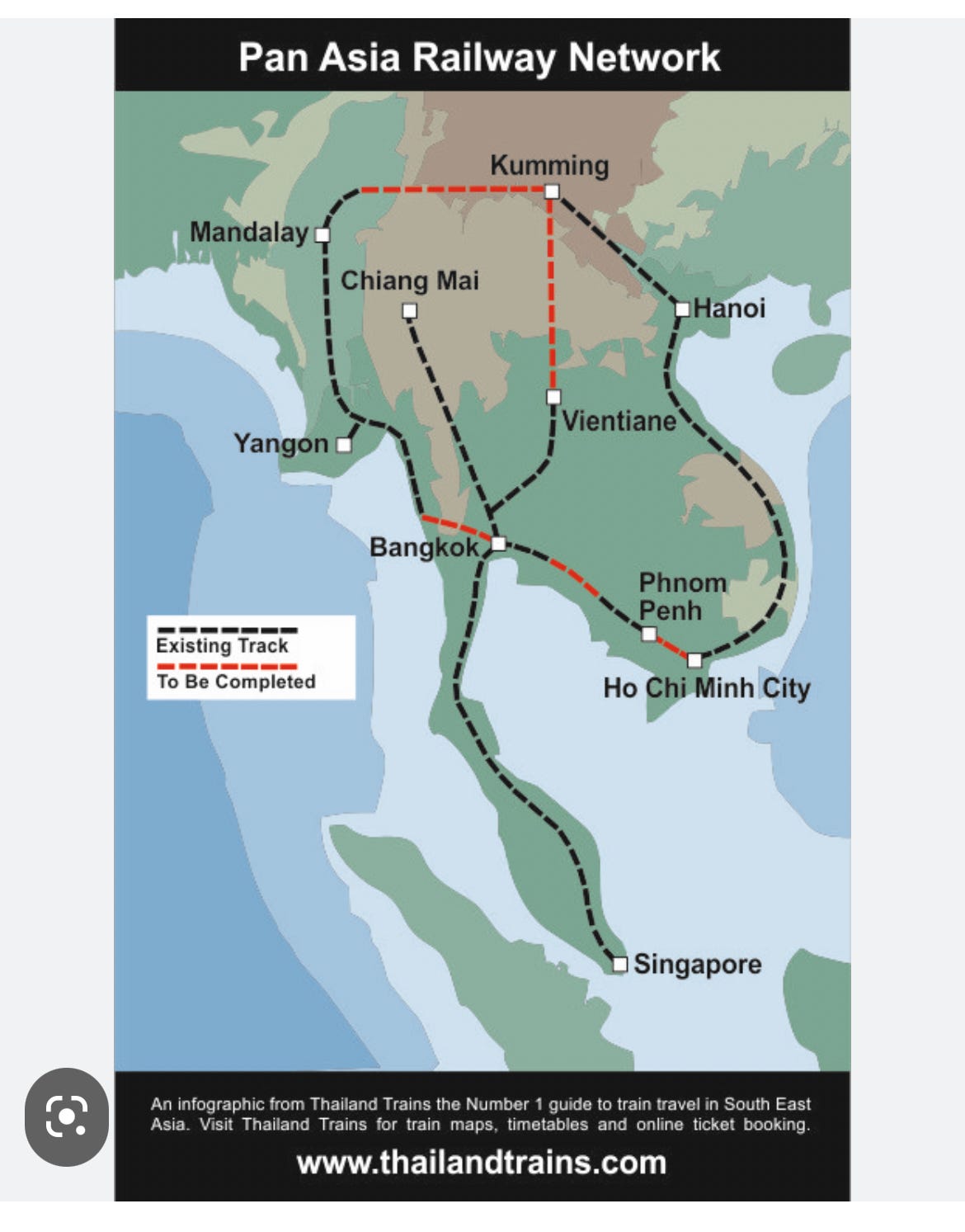The image is a highly detailed map of the Pan-Asia Railway Network, typically seen as a poster in transit hubs like subway or railway stations. It prominently displays Southeast Asia, with landmasses in shades of green and light brown, surrounded by blue water. At the top, the title "Pan-Asia Railway Network" stands out in white letters within a black rectangle. The network connects various major cities, depicted with white squares, including Mandalay, Cumming, Hanoi, Chiang Mai, Yangon, Bangkok, Ho Chi Minh City, Singapore, and more. Black dotted lines represent existing railway tracks, while red dotted lines indicate tracks planned but not yet completed, such as the connections from Cumming to Vientiane and from Ho Chi Minh City to Phnom Penh. The bottom section of the map features text that reads, "An infographic from Thailand Trains, the number one guide to train travel in Southeast Asia." It invites viewers to visit www.thailandtrains.com for train maps, timetables, and online ticket booking.